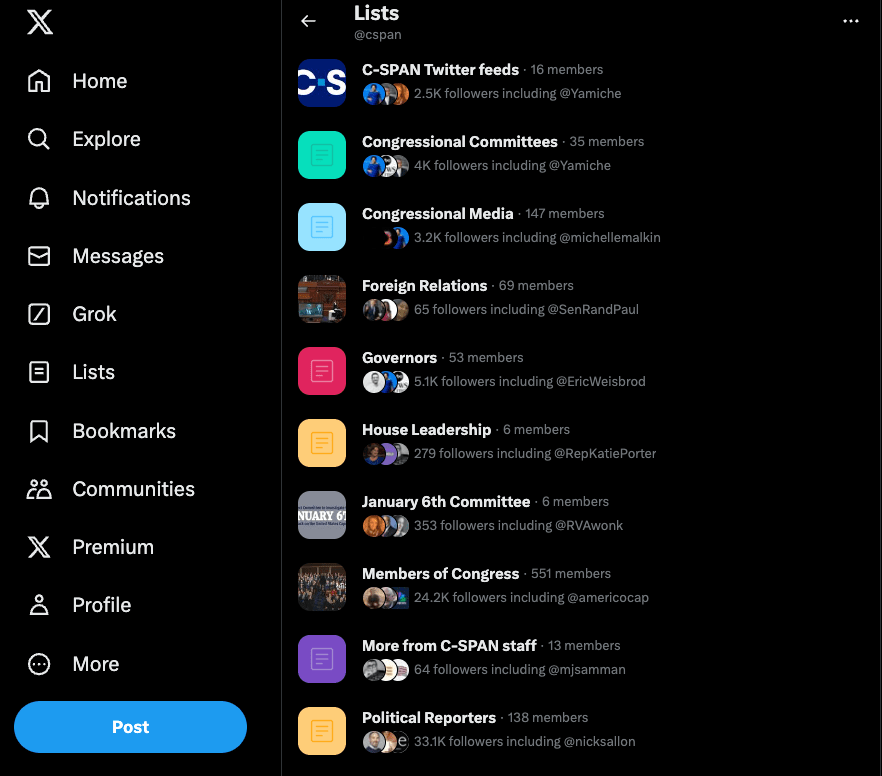The image features a dark black background with detailed elements primarily concentrated in two vertical columns.

On the left side:
- In the top left corner is the Twitter "X" icon.
- Below this icon are a series of icons with corresponding labels: 
  - A house icon labeled "Home."
  - A magnifying glass icon labeled "Explore."
  - A bell icon labeled "Notifications."
  - An envelope icon labeled "Messages."
  - A square icon with a pencil or line labeled "Grok."
  - A square icon with two lines labeled "Lists."
  - A bookmark icon labeled "Bookmarks."
  - An icon with two people labeled "Communities."
  - The Twitter "X" icon again, this time labeled "Premium."
  - An icon with a single person labeled "Profile."
  - A circle with three dots labeled "More."
- Below this list is a blue option button labeled "Posts."

On the right side:
- At the top, there is a title "Lists," followed by "@C-SPAN."
- Beneath this title are a series of blue icons with text and numerical data:
  - A blue icon with "CS" labeled "C-SPAN Twitter Feeds," indicating the number of members and followers.
  - Another blue icon labeled "Congressional Committees" with membership and follower statistics.
  - Sequentially, similar icons are presented for "Congressional Media," "Foreign Relations," "Governors," "House Leadership," "January 6th Committee," "Members of Congress," "More from C-SPAN Staff," and finally, "Political Reporters."

In the top right corner of the page:
- There are three small, evenly spaced white dots aligned horizontally.

The combination of these visual elements and labels presents a detailed overview of Twitter's functionalities and specific lists related to C-SPAN.